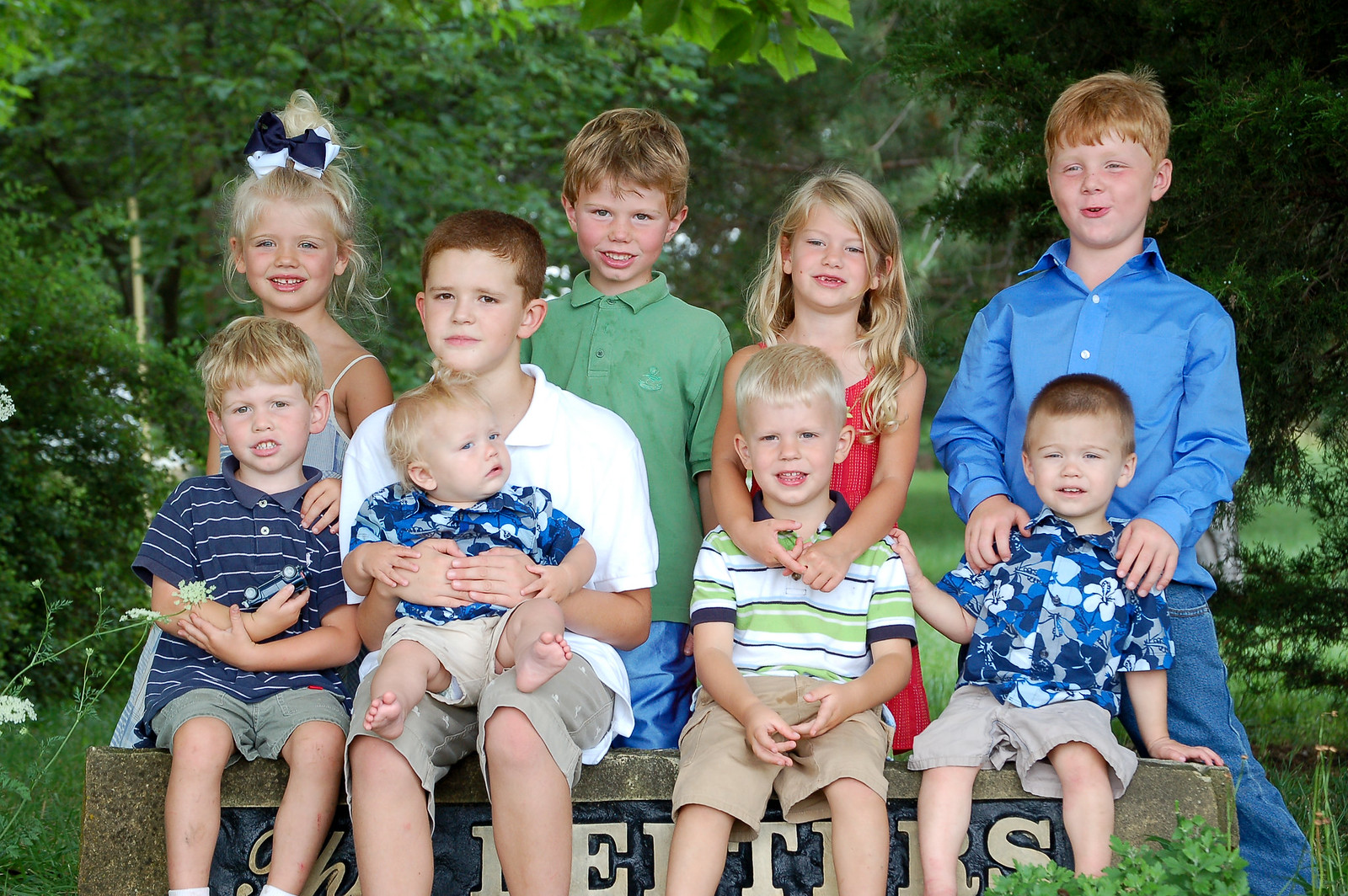This photograph captures a group of nine children seated closely together on a rectangular, concrete stone bench that bears an inscription partially obscured by their feet. The inscription, framed within a smaller dark blue rectangle with darker blue splotches, features tan lettering that includes visible letters like ‘E’, ‘T’, ‘R’, ‘I’, and ‘S’. The children are positioned in front of dark green trees, including a mix of evergreens and maples, with the maple branches extending over them. They range in age from a toddler to around ten years old. 

The eldest boy, approximately ten, is in a white short-sleeved dress shirt and gray-tan cargo pants with a small white pattern. He holds a toddler donning the same floral-patterned shirt as another boy on the far right, both wearing tan cargo pants. A girl with a strapped light gray dress and blonde hair tied up with dark blue and white bows sits to the far left. Next to her, a boy in an olive green dress shirt features short blonde and brown hair with the collar folded down. One girl, dressed in a red dress with short blonde hair, has her arms wrapped around a boy in a white and green striped shirt paired with tan cargo shorts. 

Another boy sports a dark blue floral-patterned shirt with light blue and gray flowers, alongside light gray cargo shorts and short brown hair. Behind him, a boy with short blonde hair wears a silk blue dress shirt and blue jeans, his hands resting on the floral-shirted boy’s shoulders. On the far left, a boy with a dark blue shirt with white stripes and greenish-gray cargo pants is supported by the hand of the gray-dressed girl. The serene outdoor setting, complemented by the lush greenery and the children’s varied but vibrant clothing, emphasizes a candid and warm family moment.